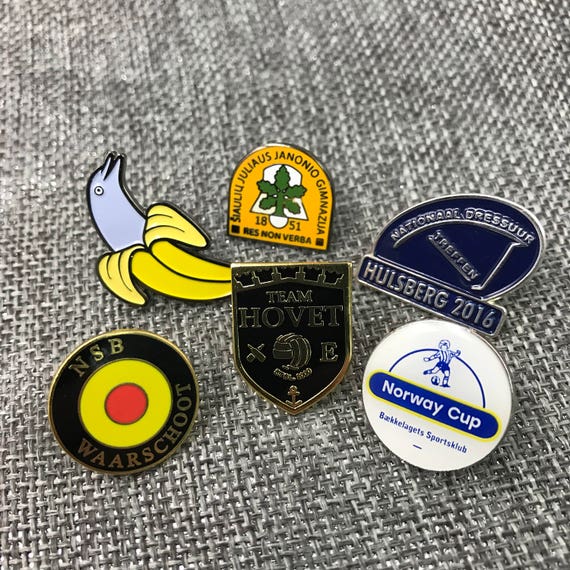The image features six small enameled pins displayed on a gray burlap, evoking a tweed-like appearance. Arranged in two rows of three, the top left pin depicts a half-peeled banana, revealing a dolphin inside instead of fruit. The top middle pin is a shield, oriented with the round part facing up, inscribed with "SIAU JULIAS JANIERO GIMNASUA," "res non verba," "1851," and an icon resembling a tree. The top right pin, dark blue with white text, reads "NATIONAL DRESSUR TREPIN" along with "HOOLSBURG, 2016," featuring a design that suggests a connection to hockey. 

In the bottom row, the left pin is a circular design with concentric rings in black, yellow, and red, marked "NSB WARSCHOOT," with the outer black ring, the yellow middle ring, and the red center resembling a bullseye. The bottom middle pin, shield-shaped with the point down, is emblazoned with "TEAM HOVET" and includes images of two crossed beer bottles, a soccer ball, the letter "E," and an anchor at the base. The bottom right pin is a white circle with blue and yellow printing, containing an image of someone kicking a soccer ball and a blue rounded rectangle with the text "NORWAY CUP," accrediting "BAKU AGETZ SPORTS CLUB."